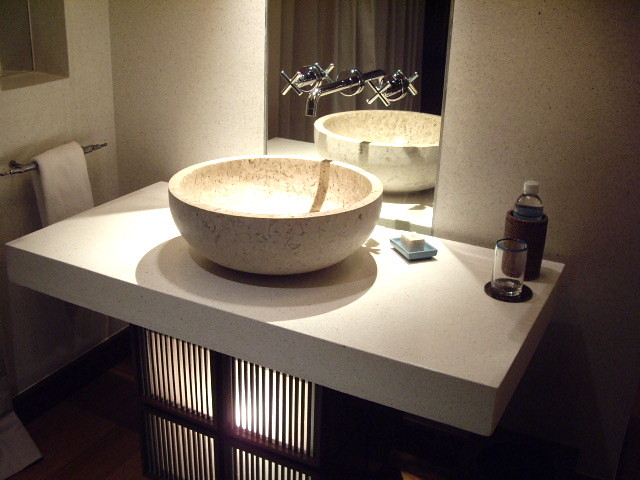The image depicts a sleek, contemporary bathroom setting, likely from a modern hotel. The centerpiece is a pedestal sink made of white composite material with subtle speckles, which is visually striking. The sink itself is a stylish vessel bowl sitting atop the pedestal, further enhancing the modern aesthetics. Uniquely, the stainless steel faucets extend directly from the mirror above, adding a sophisticated touch.

Illuminating the space, a lighted cabinet below the sink emits a soft glow through a grated effect, creating a warm and inviting ambiance. To the left, a stainless steel towel rack holds a neatly folded towel, maintaining the overall polished appearance.

On the countertop, a glass water bottle suggests this is indeed a hotel bathroom, providing guests with thoughtful amenities. The floor appears to be a rich brown color, complementing the neutral tones of the room. Reflected in the mirror, a tan shower curtain hints at the presence of a shower behind the viewer, completing the scene. Overall, this bathroom exudes modern luxury and functionality.